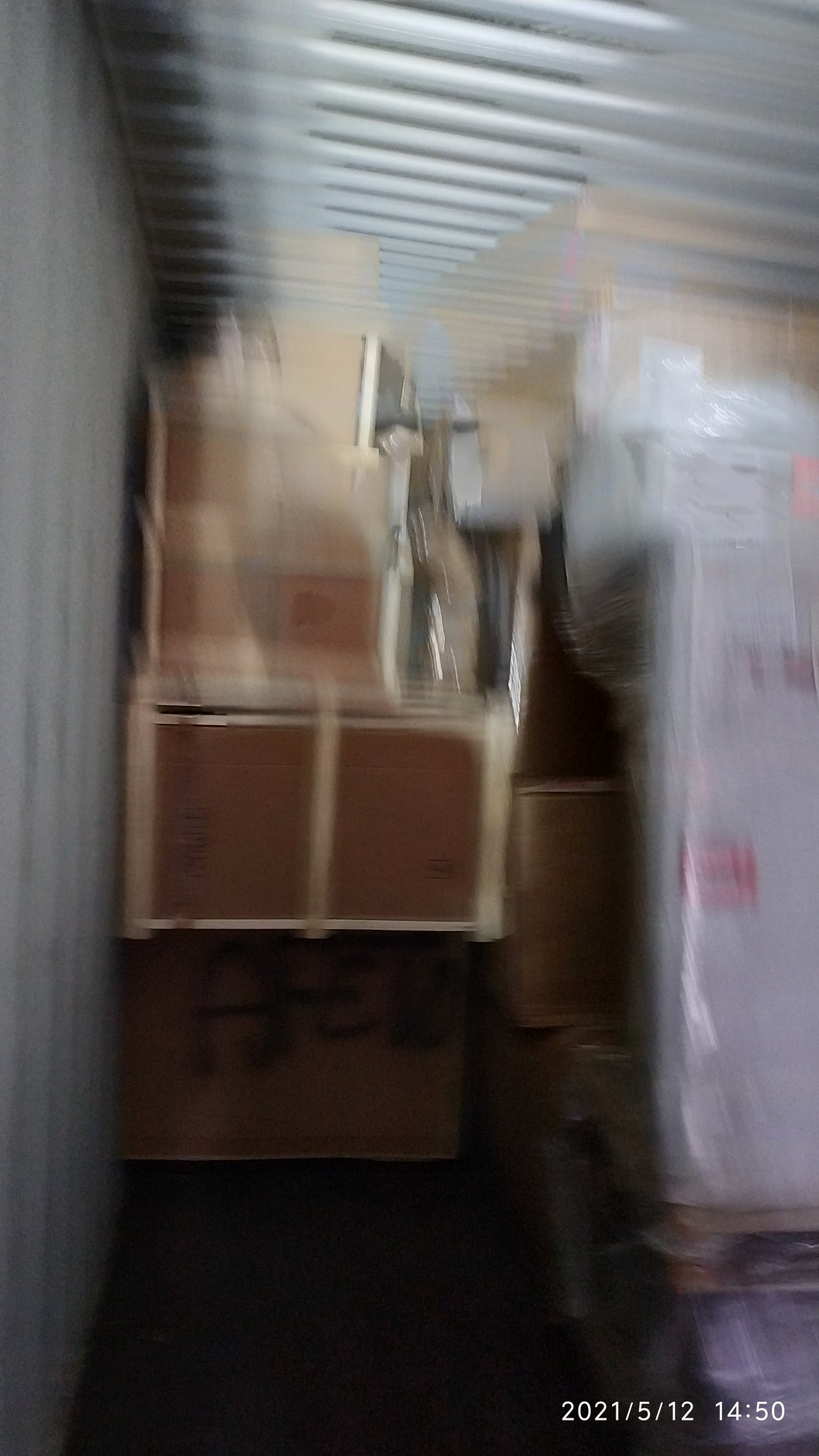A blurry photograph captures the mysterious interior of what appears to be either a semi-truck trailer or a storage shed. The left side of the image reveals a ribbed metal wall, while the ceiling follows suit with a ribbed, slanting design. Dominating the center of the scene is a tall stack of brown cardboard boxes, upon which a silverish metallic object sits prominently, its exact function uncertain due to the blur. To the right, another stack of boxes can be seen, albeit in a gray, indistinct form that suggests they might be resting on a wooden pallet. The lower right corner of the photograph is marked with a timestamp in white font, reading "2021/5/12 1450," adding context to this snapshot of an otherwise enigmatic storage space.